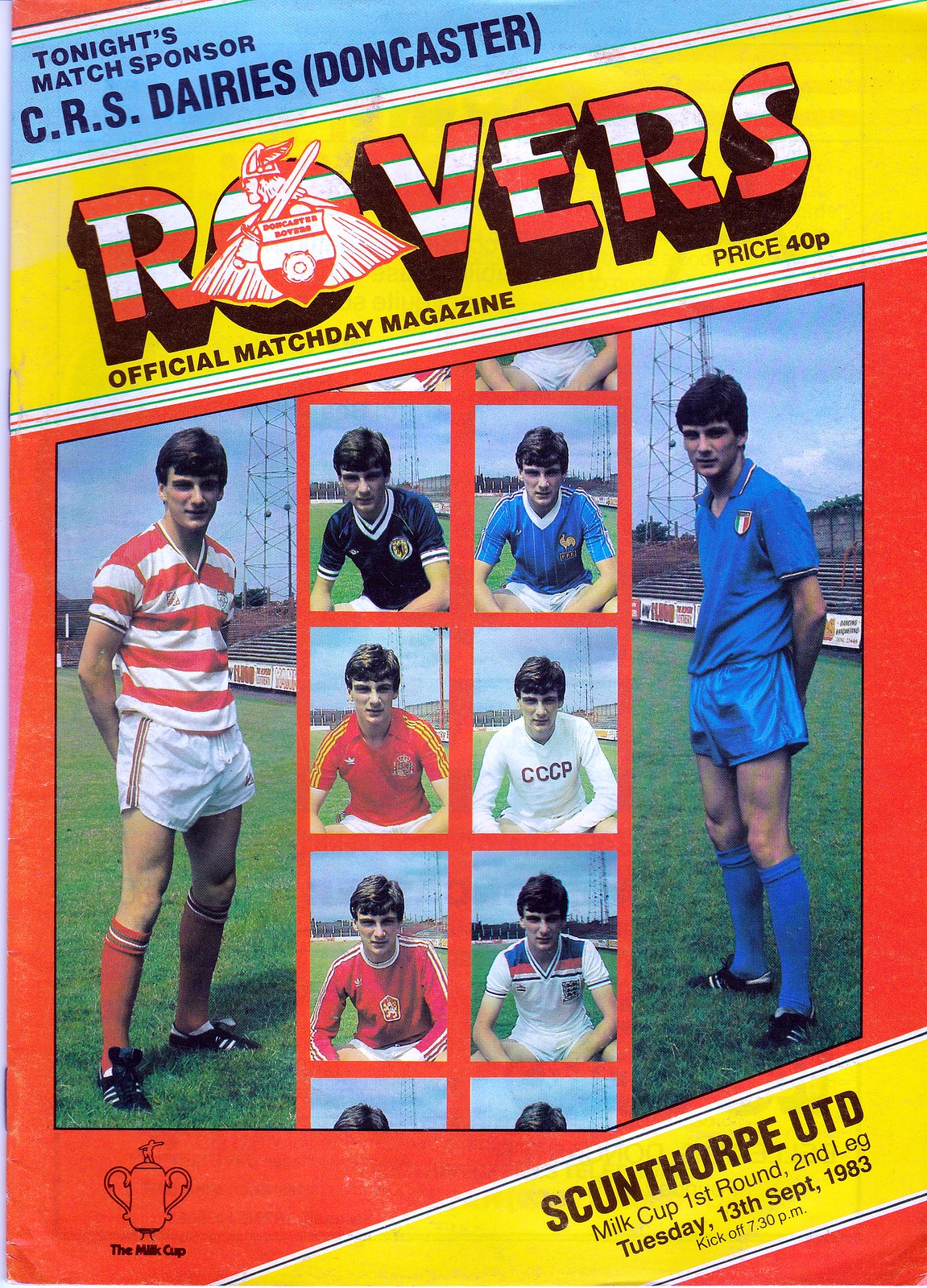This image, a tall rectangular scan of a vintage soccer magazine cover titled "Rovers Official Match Day Magazine," is mostly red and adorned with several eye-catching elements. In the upper left, a diagonal light blue stripe with white and red outlines features the text "Tonight's Match Sponsor CRS Dairies," followed by "(Doncaster)." Beneath that, bold red and white horizontal stripes spell out "Rovers," with a Viking illustration over the 'O'. 

On the lower left, it reads "Official Match Day Magazine," while the lower right notes the price, "40p." The bottom section contains various photographs and images. On the left, there's a full-body photo of a man in a red and white striped shirt, white shorts with red pinstripes, red knee-high socks, and black Adidas soccer cleats. Opposite him, on the right, is an identical-looking man wearing a completely blue uniform, appearing like an Italian jersey. 

The central band of photos features the same man in different jerseys, suggesting versatility or historical kits. The lower right includes an illustration of a trophy labeled "Milk Cup." A yellow diagonal banner across the page, from bottom left to top right, highlights "Scunthorpe UTD Milk Cup First Round Second Leg Tuesday, 13th September 1983, Kickoff 7:30 p.m." The thin white line and protruding staples on the left indicate it's a bound magazine from the 1980s.